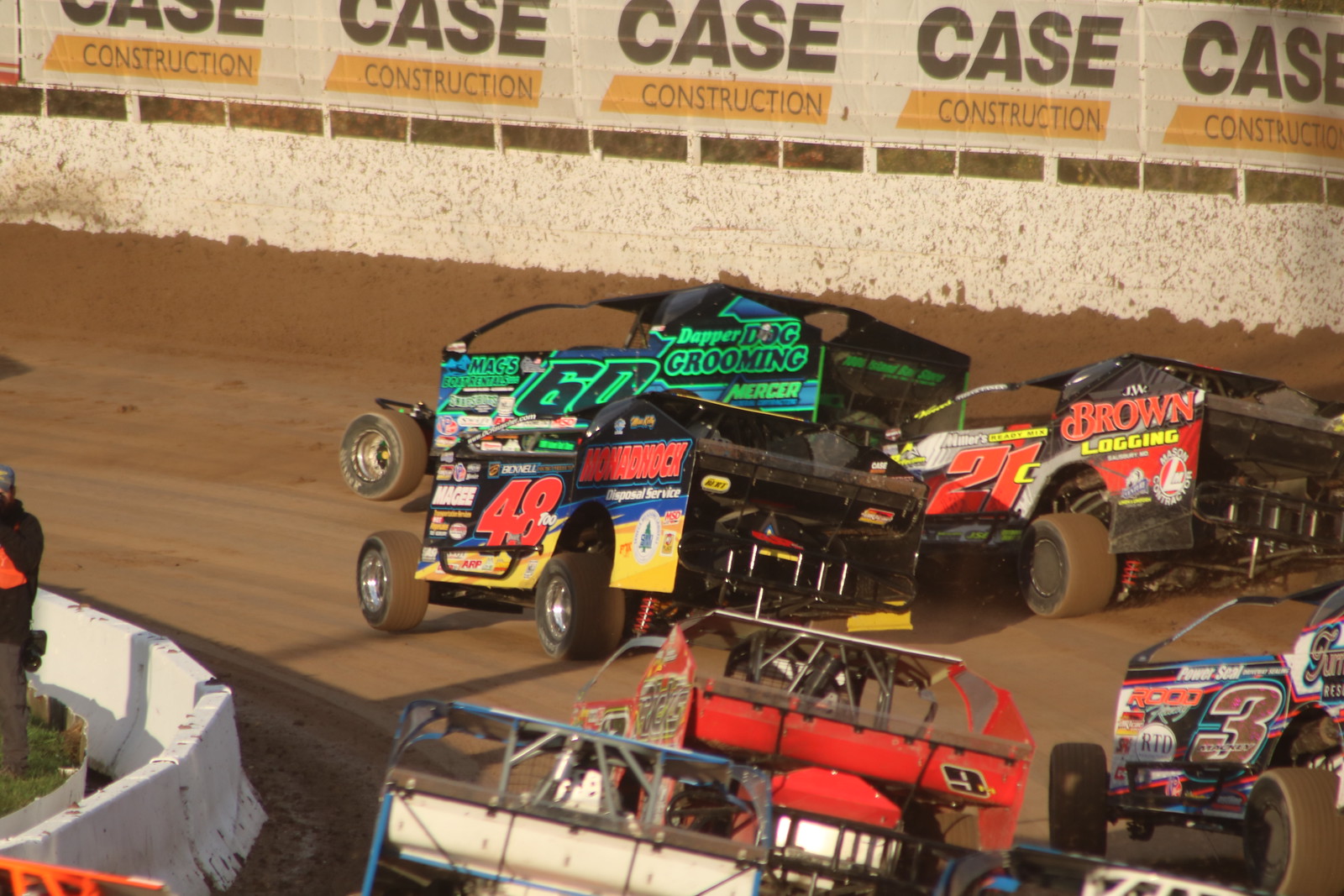The photograph captures a thrilling dirt track race featuring six specialized, open-wheel race cars in the midst of navigating a corner. These vehicles, neither traditional street cars nor F1 machines, are uniquely designed for this rugged terrain, characterized by their rudimentary, box-like bodywork adorned with numerous advertisements. As they speed around the turn, their wide tires kick up dirt and mud, showcasing the dynamic suspension keeping them grounded. 

The leading car, number 60, has a primarily greenish-black body with black or green-outlined text and is dramatically tilted to the right, with its left wheels off the ground. Directly beside it is car number 48, sporting a mostly black body with striking red text, while trailing them is car number 21 in red. The scene includes car number 3 in the lower right corner and a glimpse of car number 9 towards the back. 

In the background, a barrier with white rocks prominently displays the "Case Construction" logo, with "CASE" in bold, black capital letters and "CONSTRUCTION" also capitalized but not bold, highlighted in yellow. The dirt track is bordered by stones or barriers, adding to the gritty, high-adrenaline atmosphere of the race.